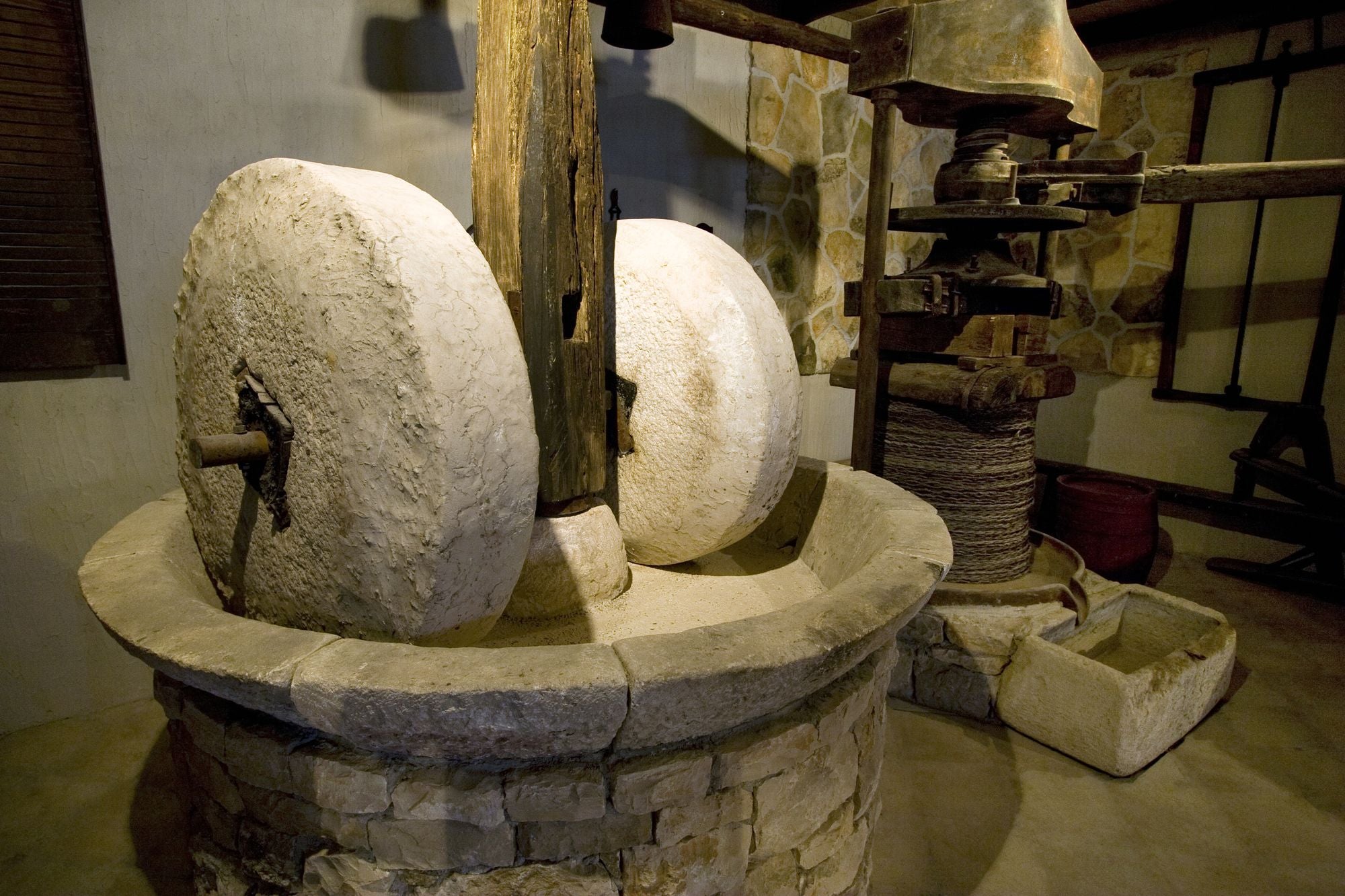The photograph depicts a meticulously restored old mill, possibly situated in a museum dedicated to antique machinery. The foreground showcases a round stone construction resembling a modern fire pit or well, featuring a stacked stone base supporting a pie pan-shaped rim. Inside the rim are two large grinding wheels, connected by an axle attached to a vertical wooden post. This setup implies a mechanism where the wheels, when cranked, would grind materials placed beneath them. 

The backdrop reveals an intricately built machine with pulleys, gears, and various metal components—presumably the drive mechanism that powers the millstones. The equipment appears well-maintained, suggesting careful restoration efforts. The walls offer a rustic ambiance, with an irregularly shaped stone wall at the back and a stuccoed or concrete wall on the left. A catch bin at the base of the machine hints at where the processed material might be collected, adding to the historic industrial charm of the scene. Attached copper pipes and other hardware contribute to an overall intricate and functional design.